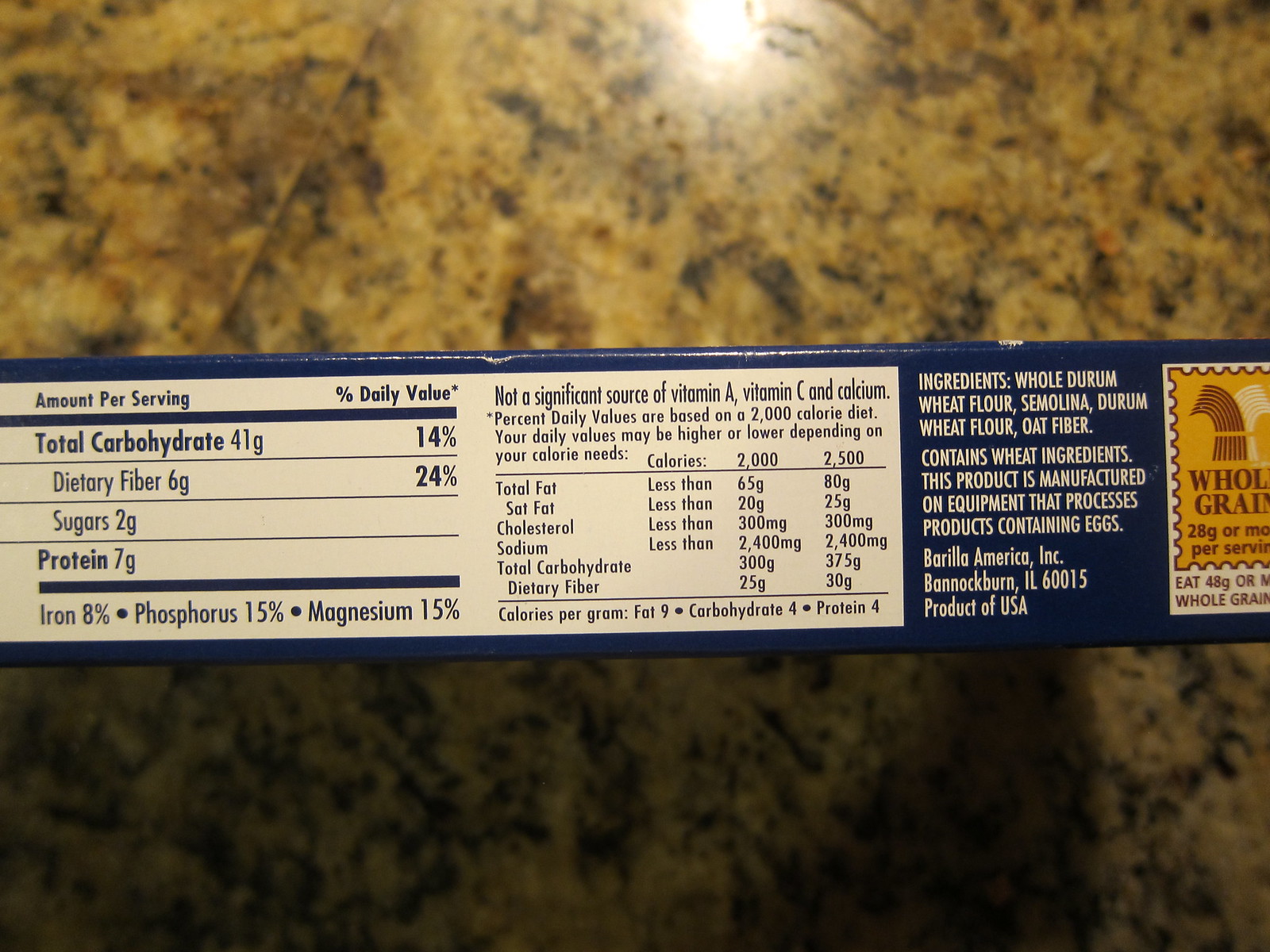The photograph captures the side of a box of pasta, specifically spaghetti, set against a dark brown, granite-like surface that has a matte finish with subtle reflections of light at the top. The dark blue label on the box prominently features vital details about its nutritional value and ingredients. To the left of the label, you can find the nutritional facts, which include 14% total carbohydrates, 24% dietary fiber, 2 grams of sugar, and 7 grams of protein per serving. Additionally, it lists essential minerals such as iron, phosphorus, and magnesium. On the right side, the ingredients are printed in white, specifying whole durum wheat flour, semolina, oat fiber, and noting that the product contains wheat ingredients. It also mentions that it is manufactured on equipment that processes products containing eggs. The manufacturer is Borrella America Inc., and the product is made in the USA. A yellow sticker towards the right side of the box clearly indicates that the product is made from whole grains, making it a nutritious choice suitable for purchase in a retail store.